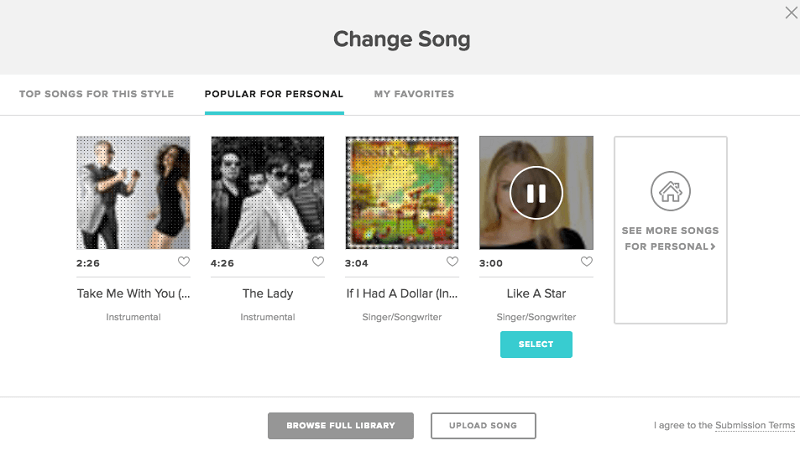The image depicts a music-related website interface. At the top, a gray bar labeled "Change Song" in black text is accompanied by an 'X' icon for closing the bar. Below it, a white bar features categories such as "Top Songs for This Style," "Popular for Personal," and "My Favorites." 

The first album cover displays a man and a woman dancing, alongside the title "Take Me With You (Instrumental)," with a duration of 2 minutes and 26 seconds. Next to it, an album cover with four men wearing sunglasses is labeled "The Lady (Instrumental)," lasting 4 minutes and 26 seconds. 

The third cover is pixelated and appears to depict animals dancing, titled "If I Had a Dollar," with a duration of 3 minutes and 4 seconds, categorized under singer-songwriter. Finally, an album featuring a blonde woman with a visible pause button bears the title "Like a Star," also under singer-songwriter, with a duration of 3 minutes. 

Options to "Select" and "See More Songs for Personal" are available, followed by buttons labeled "Browse Full Library" and "Upload Song."